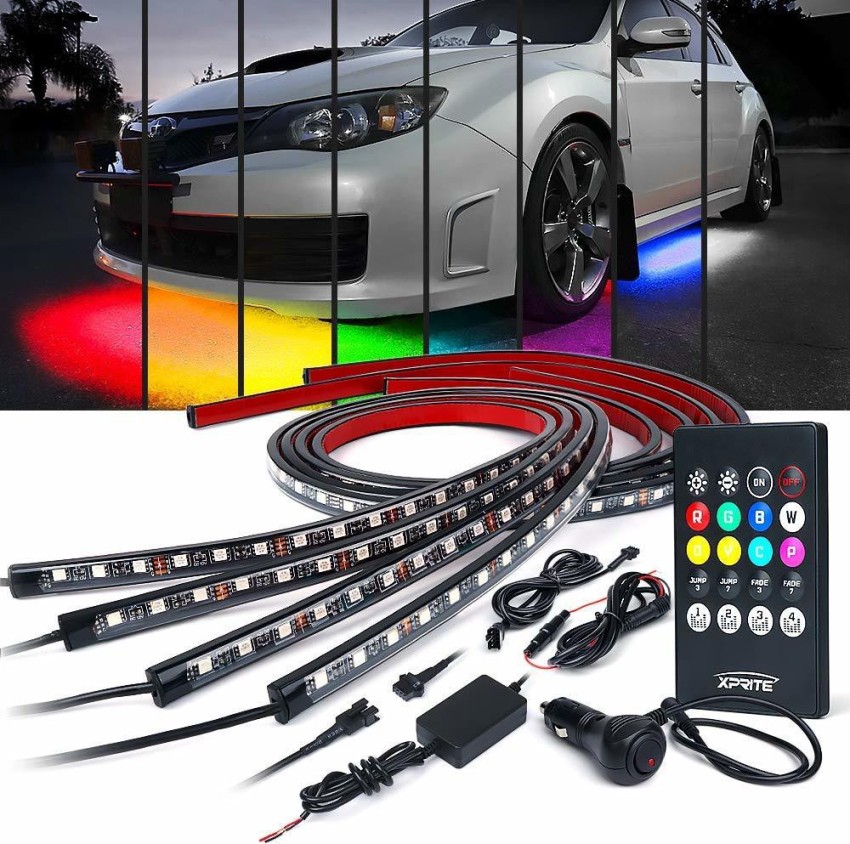This image is an Amazon product listing for underglow LED lights designed for vehicles. At the top, there's a white Subaru showcasing the rainbow-colored lights projected onto the ground beneath it. The lights are arranged in a spectrum from red on the left, followed by orange, yellow, green, light blue, purple, and dark blue towards the right. The vibrant rainbow extends along the car's front fender, highlighting its undercarriage against a gray ground and green trees in the background. Below this display, the actual product is featured - four LED light strips with connecting wires, a cigarette lighter plug for power, and a remote control. The remote, detailed in the lower right corner, includes an on/off button, multiple color buttons, and numbered buttons for various functions. The light strips are displayed coiled, with black connecting cords and adhesive backs for easy installation. This comprehensive setup allows for customizable vehicular underglow, enhancing the car's aesthetic appeal.